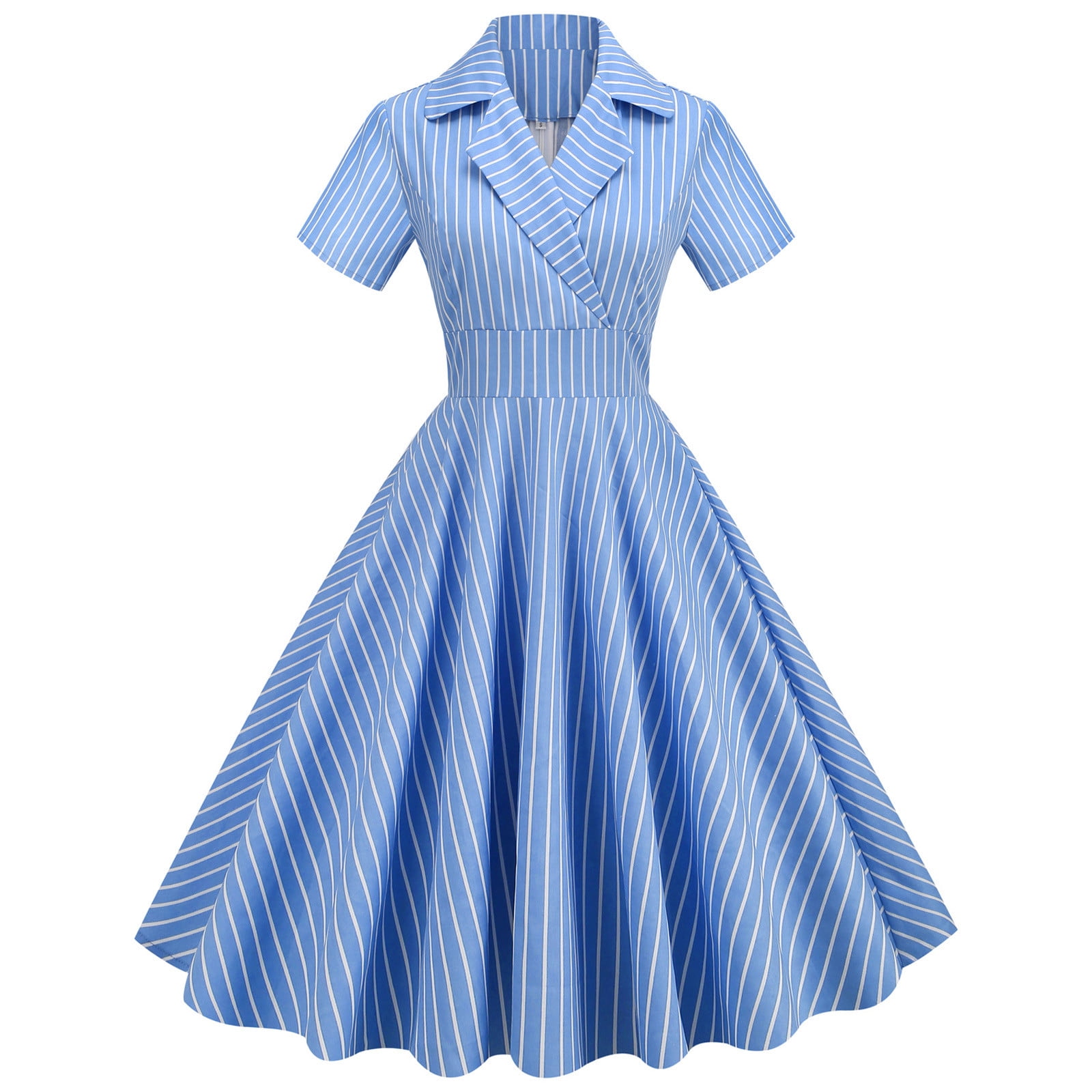This image resembles a product photo commonly seen on online shopping platforms like Amazon, featuring a vintage-inspired, 1950s-style dress against a completely white background. The dress is not worn by a model or displayed on a mannequin, making it the sole focus of the image. It is a light blue, collared, short-sleeve dress adorned with vertical white pinstripes. The design has a form-fitting cut through the torso, accentuated by a slender waistband, before flaring out into a bell-shaped skirt that falls just below the knee. The dress embodies a classic, old-fashioned look, with details reminiscent of attire worn by housewives or diner waitresses from the 1950s. The white background emphasizes the simplicity and vintage charm of the dress, highlighting its rich baby blue color and delicate pinstriped pattern.